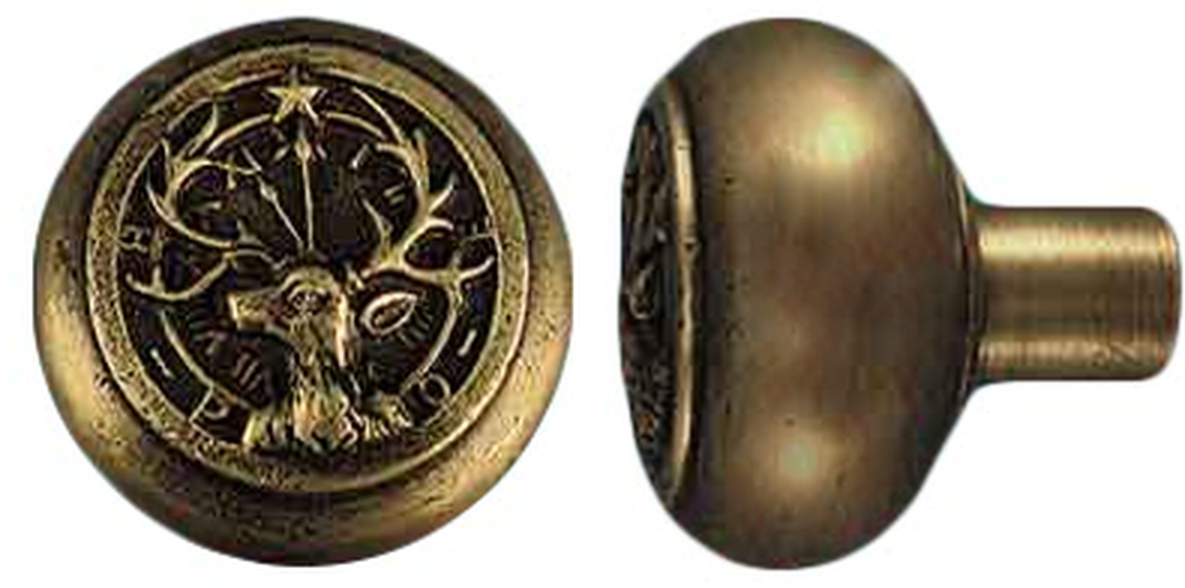The image showcases two detailed views of brass doorknobs, cylindrical in shape with a smooth, spherical surface, tapering to a thin connecting tube visible in the side view. The front of the doorknob, prominently displayed on the left side of the image, features an intricate etching of an elk's head, gazing leftward. This elk is adorned with two antlers curving towards each other, connected by a line leading to a central five-point star. The decorative elements are etched in a golden brown hue, giving the doorknob an antique, stylized appearance. The background is white, highlighting the doorknob's detailed craftsmanship, making it a distinguished piece among door hardware and accessories, potentially valued as a vintage construction material.